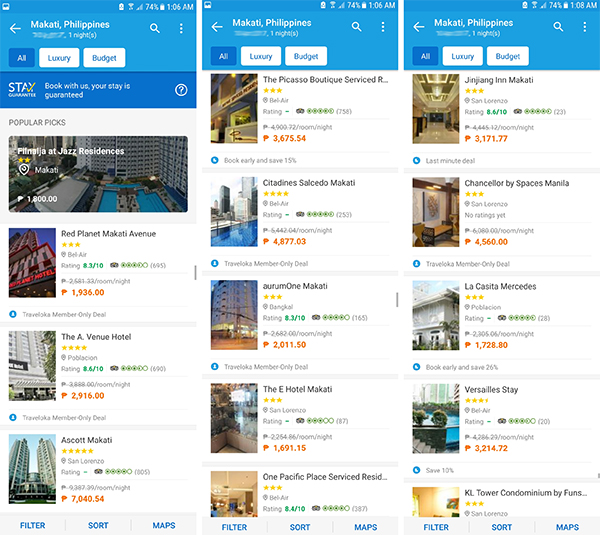The image showcases three vertical, side-by-side screenshots, presumably from a cell phone, each taken at slightly different times. They illustrate a search for hotels in the Philippines on a Google platform via an Android phone. The screenshots are almost identical in layout, featuring lists of various hotels, each accompanied by a photograph, the hotel's name, the nightly price in Philippine pesos, and a star rating.

Across all three screenshots, the user has opted to display both luxury and budget options, evidenced by the selection of the "All" button. The screenshots have a clean, white background, further emphasizing the neat presentation of the hotel listings. The consistent elements across the screenshots suggest they were taken within a short time span: the two on the left show the time as 1:06 AM, while the one on the right shows 1:08 AM. The battery indicator in all three displays 74% charge.